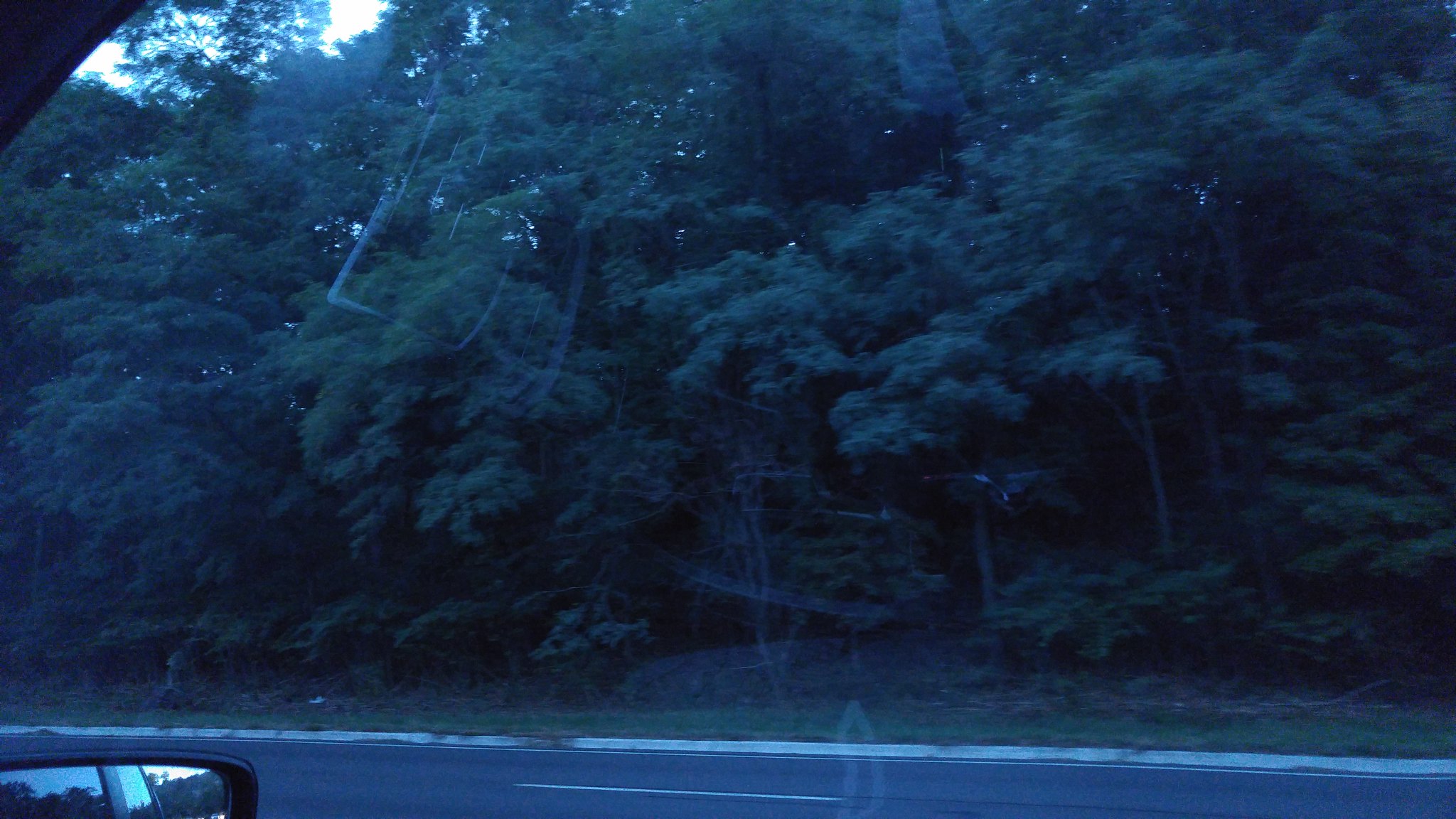A scenic view from inside a vehicle captures a serene off-street area blanketed with tall, bushy trees. The street is visible through the vehicle's windshield, including a distinct road line running through it. The bottom left-hand corner of the image features a partial glimpse of the rearview mirror, which subtly reflects part of the interior and a faint image of the surroundings. The top of the frame is adorned with bright patches of sky, peeking through the dense foliage, adding a touch of luminance to the overall green expanse. The abundant trees, with their lush and vibrant green leaves, tower majestically, creating a peaceful and immersive natural setting.